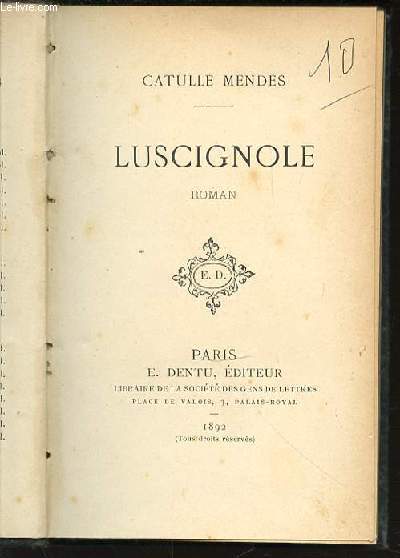The image features a close-up view of an aged book, likely a French play or literary work, as indicated by repeated mentions of cues and names associated with Paris. The page appears to be an inside cover or an opening page, showcasing a worn, tan surface with predominantly black text that reads, "Luz Cigonoli" and "Roman" among other words. The phrase "Cthulhu Mendes" is also visible, albeit with less certainty about its exact placement. Additional text includes "Paris" and a publication year of "1892." The book's age is evident from the faded and discolored page, hinting at a vintage quality. An emblem bearing the initials "E.D." is centered on the page. This overhead shot of the book suggests that it might be laying on a table, potentially being studied by someone rehearsing lines, perhaps in preparation for a play.